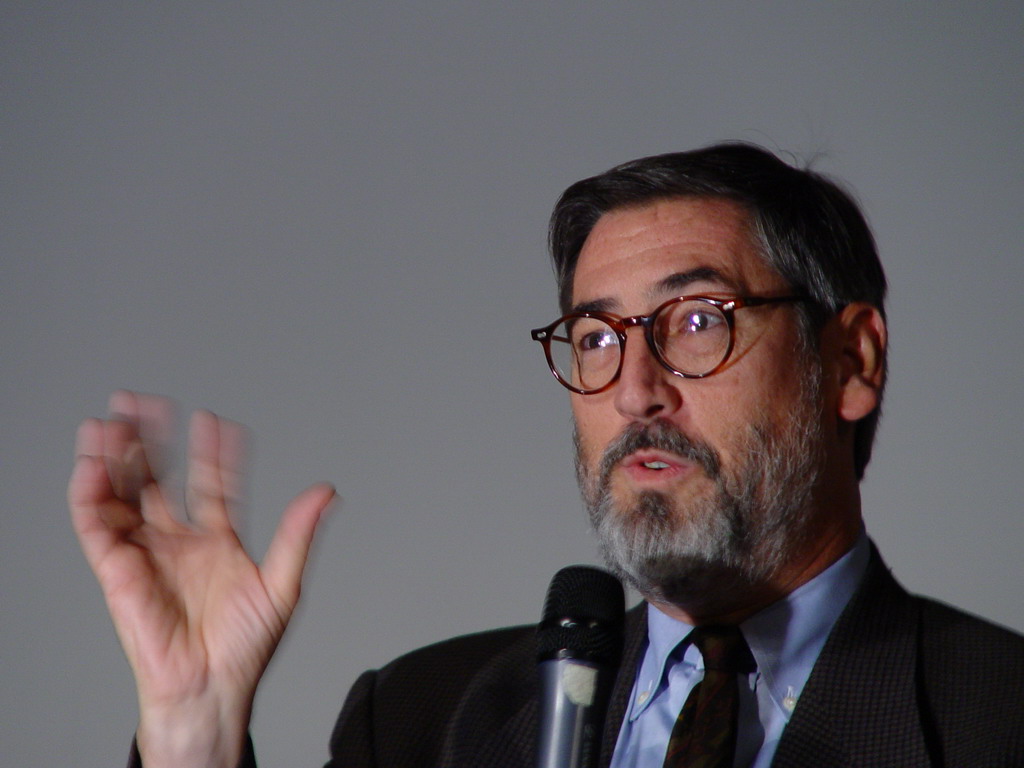The detailed color photograph captures a close-up view of American actor and director John Landis as he delivers a speech. The background is a plain gray wall, providing contrast to his figure. Landis is captured in mid-sentence, holding a microphone with a black grill and silver handle partially cut off at the bottom of the image. His thick mustache, accompanied by a graying beard and sideburns, frames his expressive face. His hair, a mix of dark brown with some gray, is cut short. His distinctive tortoise-shell round glasses, reflecting some bright lights, add a characteristic touch. He is dressed in a textured, square-patterned black suit, complemented by a light blue dress shirt with a collar and a dark blue or brown tie. His right hand is raised in a gesturing motion, slightly blurred to indicate movement as he emphasizes a point.